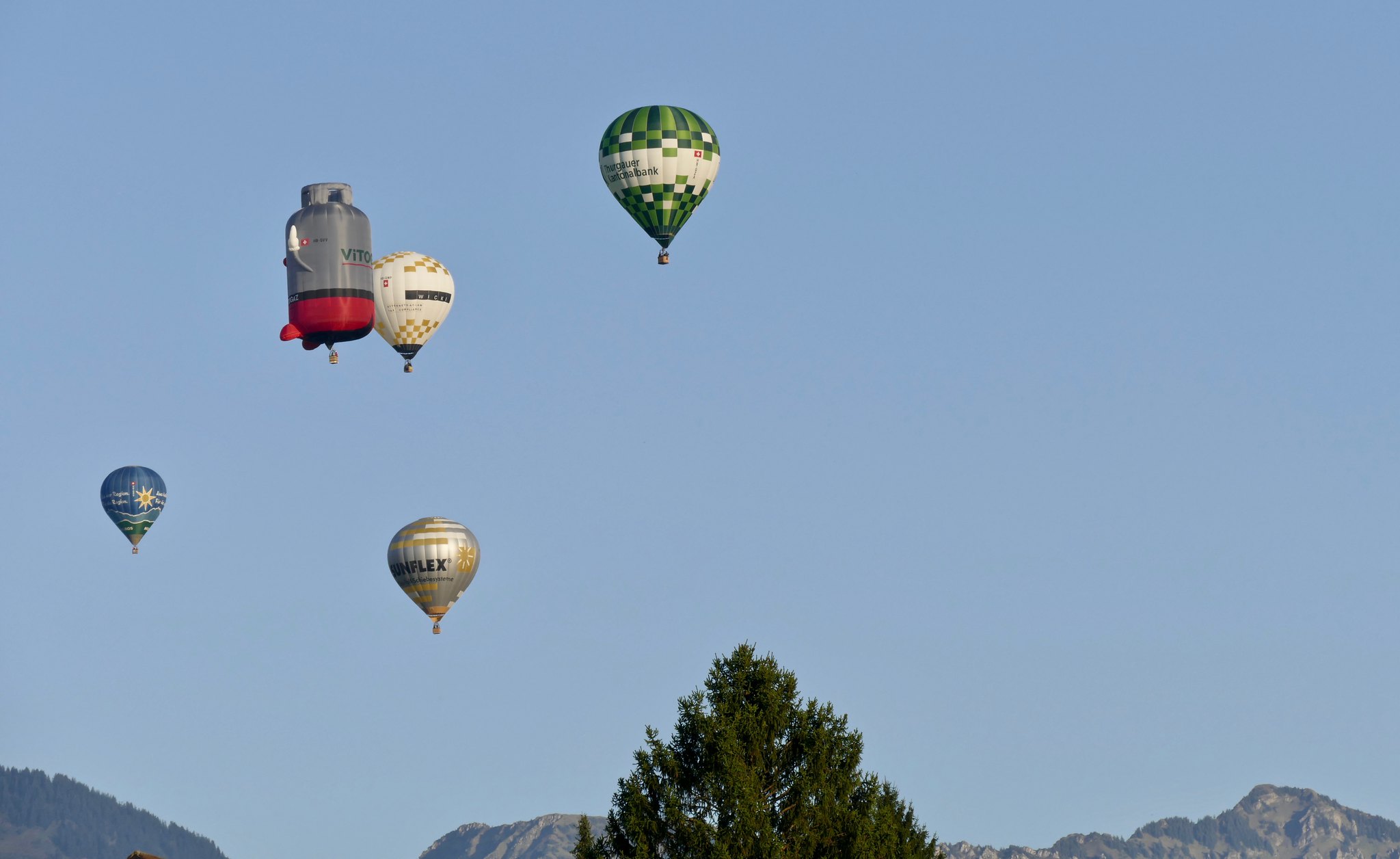This color photograph captures a clear blue sky with five hot air balloons drifting across it, all positioned to the left of the image's center. The bottom quarter of the image shows the tops of mountains and a prominent tree in the foreground, reaching up about a fourth of the picture. The balloons are detailed as follows, from left to right: the farthest balloon is blue with a sun artwork; the next one, slightly closer, is metallic silver and gold; above these are two balloons close together, one resembling an alcohol keg or canister in gray-red, and the other having a golden and white checkerboard pattern; the nearest balloon features a green checkerboard design with a white and cream stripe across the middle. The image is landscape-oriented and, while the background is slightly grainy, the vibrant colors and unique shapes of the balloons stand out beautifully against the clear sky.